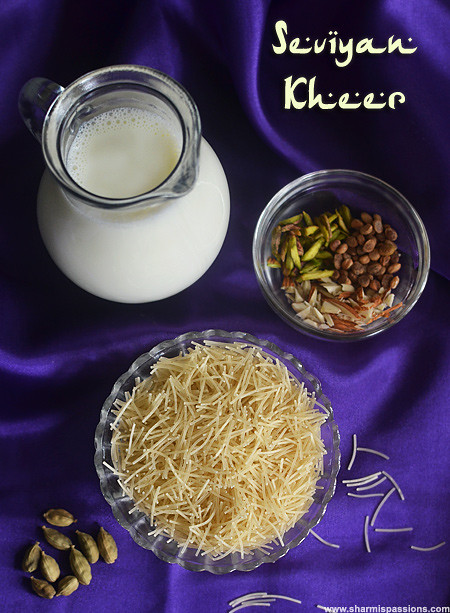In the image, a variety of foods are artistically arranged on a luxuriously draped purple cloth, which resembles a silky tablecloth with a slightly ruffled texture. Dominating the upper left portion is a glass pitcher filled with milk, oriented with the handle toward the upper left and the spout toward the lower right. Adjacent to this, a smaller glass bowl contains an assortment of grains and other morsels, including what appears to be sliced almonds and possibly some green items and protein pieces. Near the center bottom of the image sits another bowl filled with what looks like shredded cheese or perhaps cut-up noodles, with additional similar noodles scattered outside the bowl on the cloth. In the bottom left corner, a small collection of beans is visible. At the top of the image, text spelling "SEVIYAN KHEER" is displayed, accompanied by some dots, suggesting it might be in a foreign script. At the bottom, though slightly blurry, the URL "www.charmiapassions.com" is seen, hinting at a possible source or context for the meal. The overall composition suggests that the various ingredients are intended to be used together in a culinary creation.